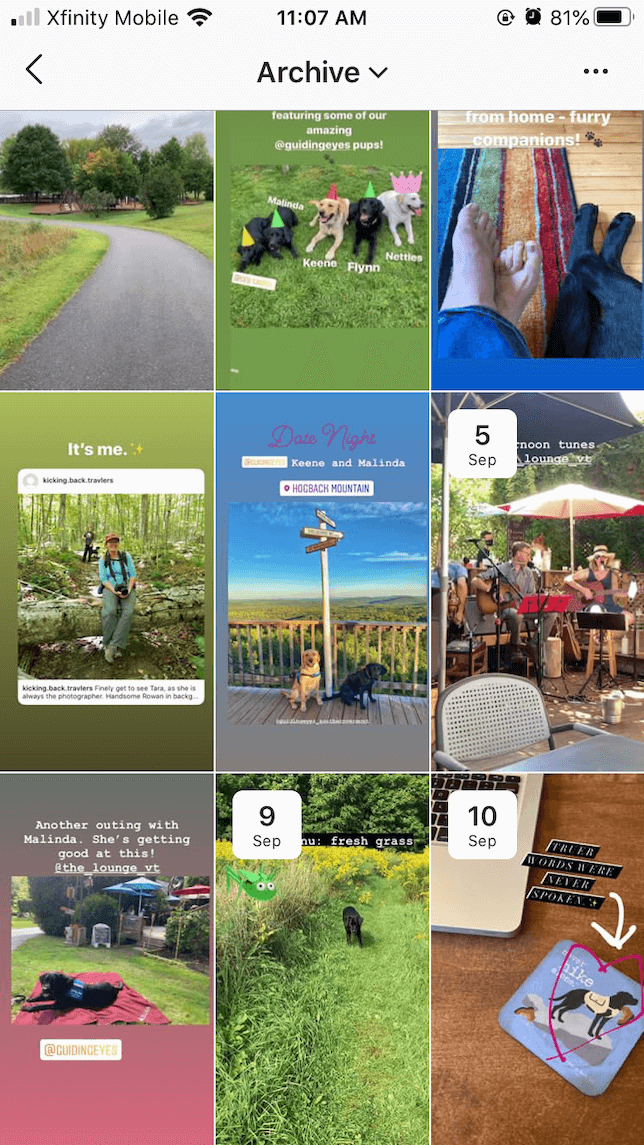This image is a detailed screenshot displaying someone's photo collection on a mobile device. Starting from the top, the status bar reveals full signal strength, the carrier Xfinity Mobile, a Wi-Fi connection, and the time, 11:07 AM. Moving to the right side of the status bar, it shows icons for an active alarm, 81% battery life, and other notifications.

The main section of the screen labels the collection as "Archive," featuring a grid of nine photos arranged in three rows and three columns. Here's a breakdown of each image:

1. **Top Left:** A road or driveway flanked by green grass and trees.
2. **Top Center:** Four or five dogs wearing birthday hats, lying in the grass. Some unreadable text accompanies the image.
3. **Top Right:** A photographer’s point of view capturing their legs and the person next to them, focusing on their feet.
4. **Middle Left:** Titled "It's me," showing a person sitting on a log, likely during a hike.
5. **Middle Center:** Labeled "Date Night," featuring two dogs.
6. **Middle Right:** Marked with "September 5th," showing a group of people on a patio.
7. **Bottom Left:** A dog resting on a mat in the grass with the caption "Another outing with Melinda, she's getting good at this," tagging someone.
8. **Bottom Center:** Dated "September 9th," depicting a dog in a field or grassy area.
9. **Bottom Right:** Labeled "September 10th," the image shows a corner of a laptop and a cardboard coaster featuring a picture of a dog, with some unidentifiable text.

Each photo includes specific dates or titles hinting at the context, such as outings, personal moments, and special occasions with pets.